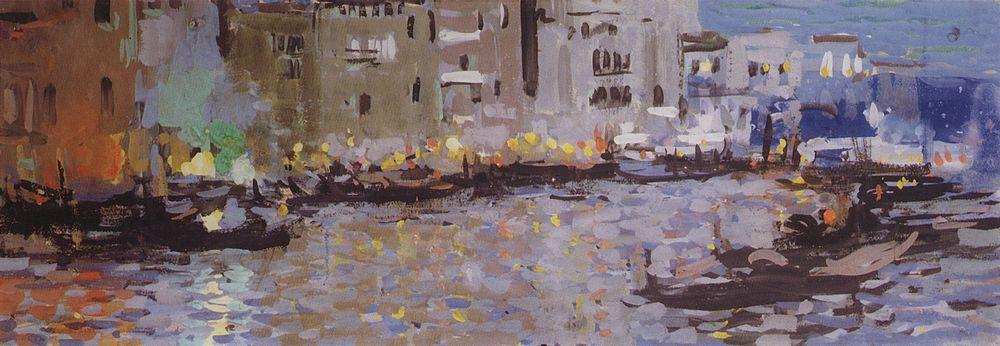The image depicts a long, horizontal painting in the Impressionist style, primarily using oil paint. The scene is set along a riverfront, canal, or another body of water, and showcases a distinctly European cityscape as a backdrop. The water is richly dappled with an array of colors, including oranges, yellows, golds, blues, and whites, reflecting the various lights and the sky. Several boats populate the water, appearing in shades of brown and tan. The buildings in the background are a mix of orange, brown, tan, off-white, and gray tones, painted with a deliberately smudged and imprecise technique that is characteristic of Impressionism. The buildings on the left side lean more towards orange and brown hues, while those on the right are predominantly blue and gray. The image suggests an evening setting, with lights casting orange and yellow reflections on the rippled water. Additional lights, possibly from lamp posts, are faintly visible against the sky in the background, enhancing the scene's atmospheric depth.